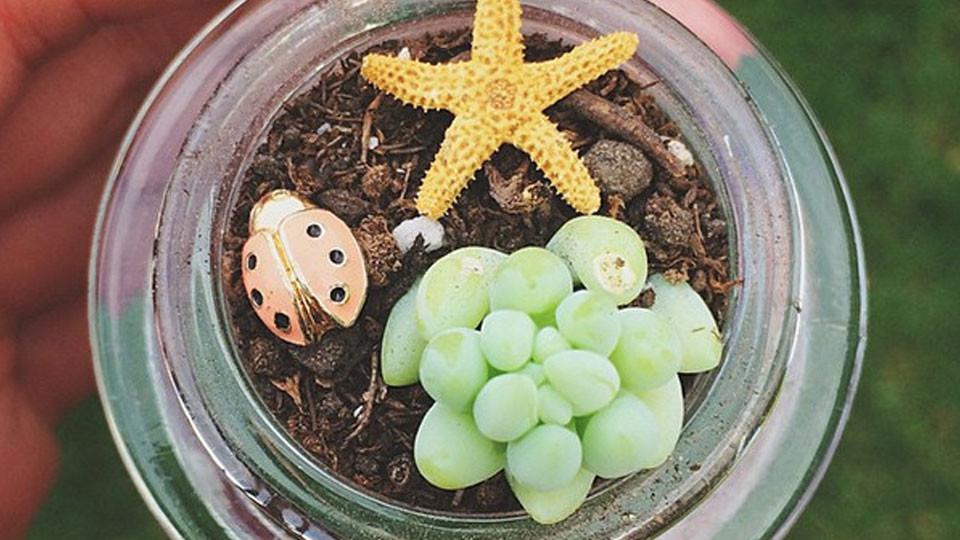The photograph presents a close-up, overhead view of a glass jar occupying the entire frame. Inside the jar is a composition of natural and artificial elements set against a backdrop of dirt and sticks, evoking an outdoor environment. Predominantly brown tones represent the earth materials. At the top of the jar rests a yellow starfish, drawing immediate attention. Below, a cluster of green, round objects reminiscent of either a cactus or grapes adds an intriguing element. To the left, a toy ladybug, distinctive with its gold head, brown wings, and black spots, adds a whimsical touch. The scene is devoid of any textual elements, focusing purely on the eclectic assortment within the jar.